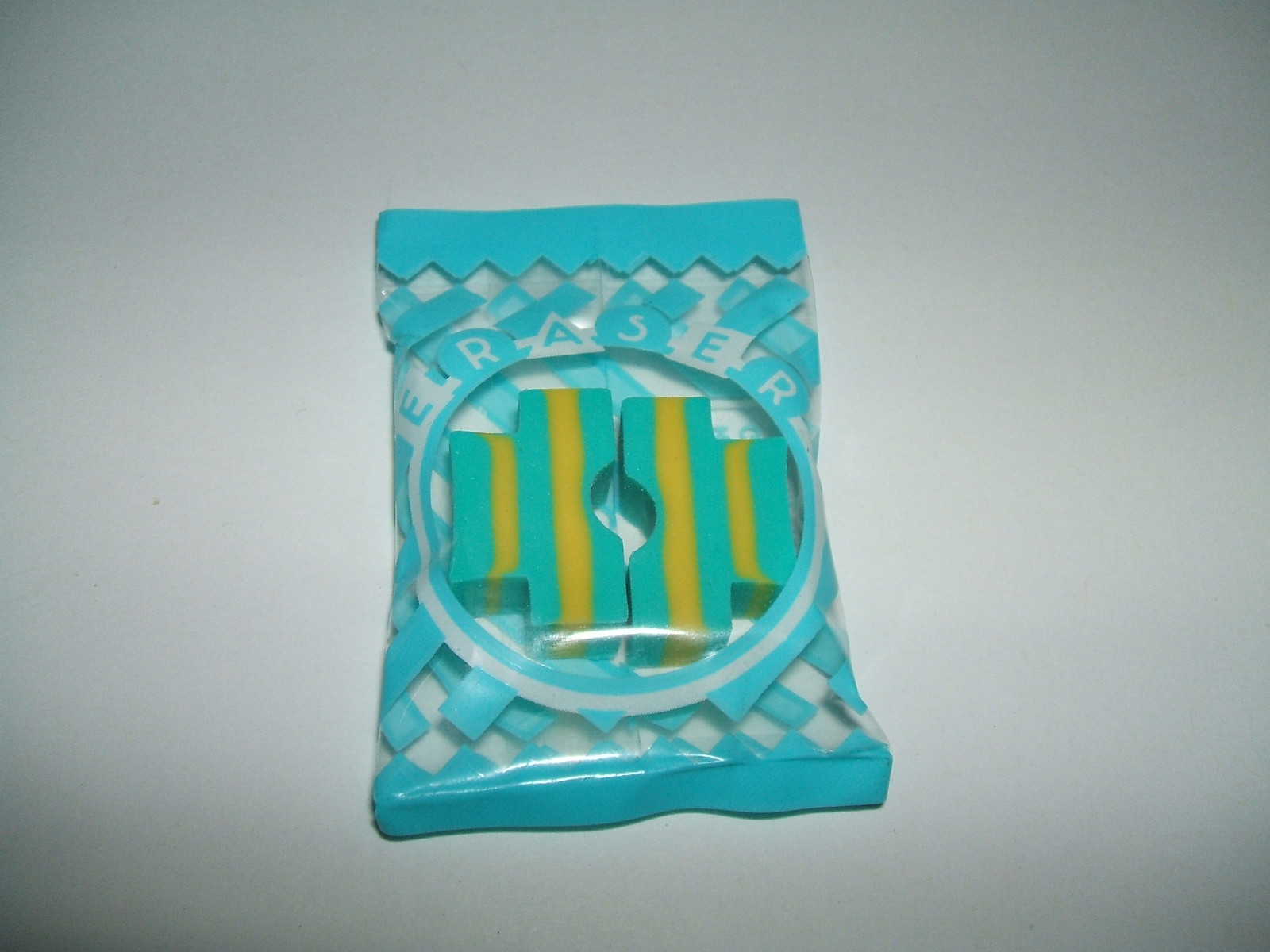The image depicts a turquoise-blue plastic package of erasers, positioned almost centered on a gray-white surface, possibly a table. The package is adorned with a jagged design on both the top and bottom edges. In the middle of the package, there is a transparent circular window displaying the two erasers inside. Each eraser is a powder blue or greenish color with vertical yellow stripes. The word "ERASER" is prominently written on the package, with the lettering primarily in blue, except for the R's and the S, which have a blue background with white letters. The photograph captures the unopened package in a straightforward manner against the neutral background.